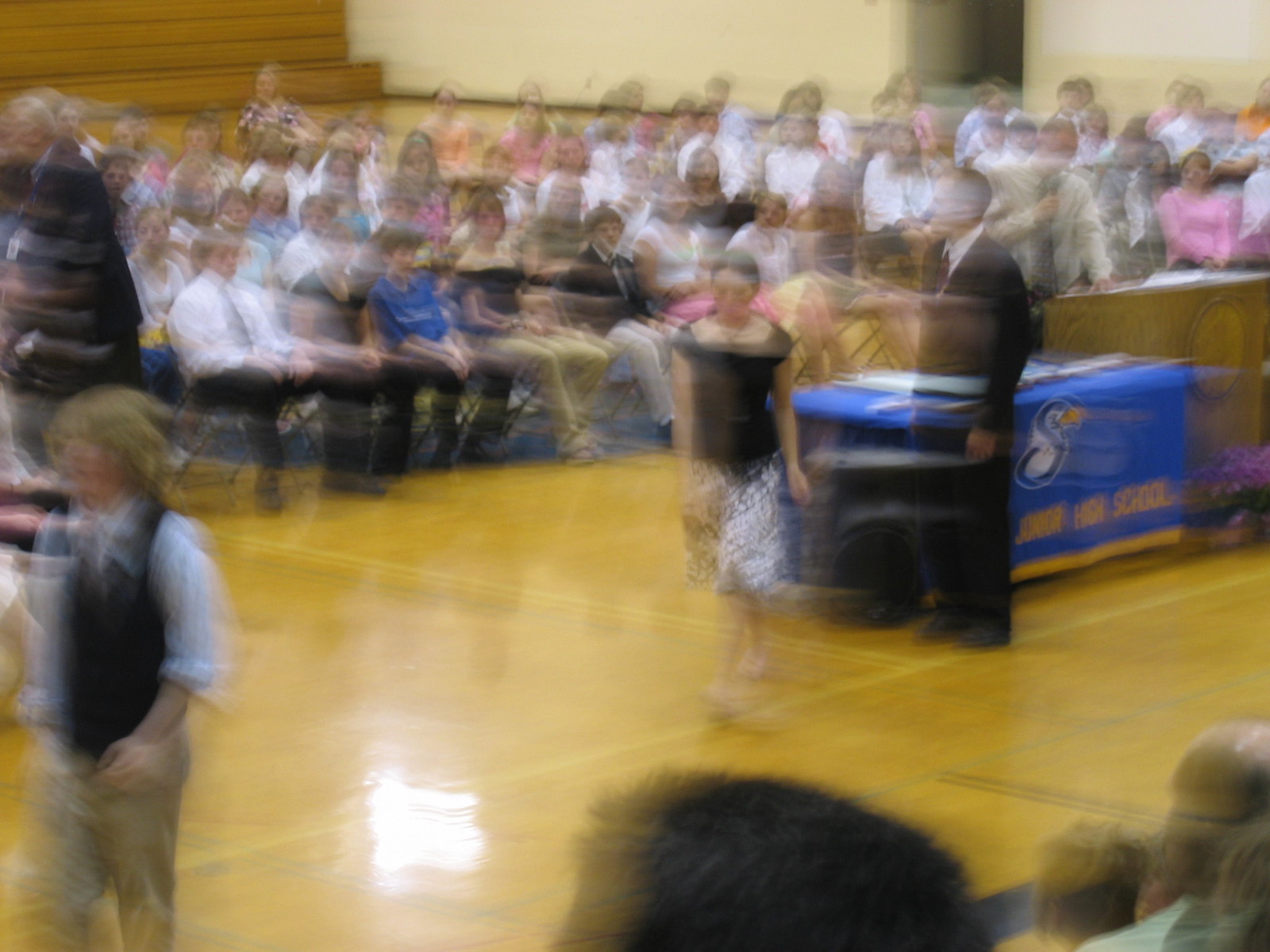In this blurry image, a school gymnasium serves as the backdrop for what appears to be a formal event. Rows of chairs, neatly arranged, accommodate both students and adults, all dressed in formal attire. The young men are notably wearing ties, adding to the formality of the occasion. At the front of the audience stands a table draped in a blue and gold tablecloth, emblazoned with the words "High School" in gold lettering. Beside this table sits a man in a black suit, white shirt, and tie, possibly an authority figure or guest speaker. To the left of the image, two students—a boy and a girl—are captured walking away from the man, possibly having just received an award or recognition. The overall scene suggests a celebratory event, possibly a graduation or an awards ceremony, taking place in a high school gymnasium.